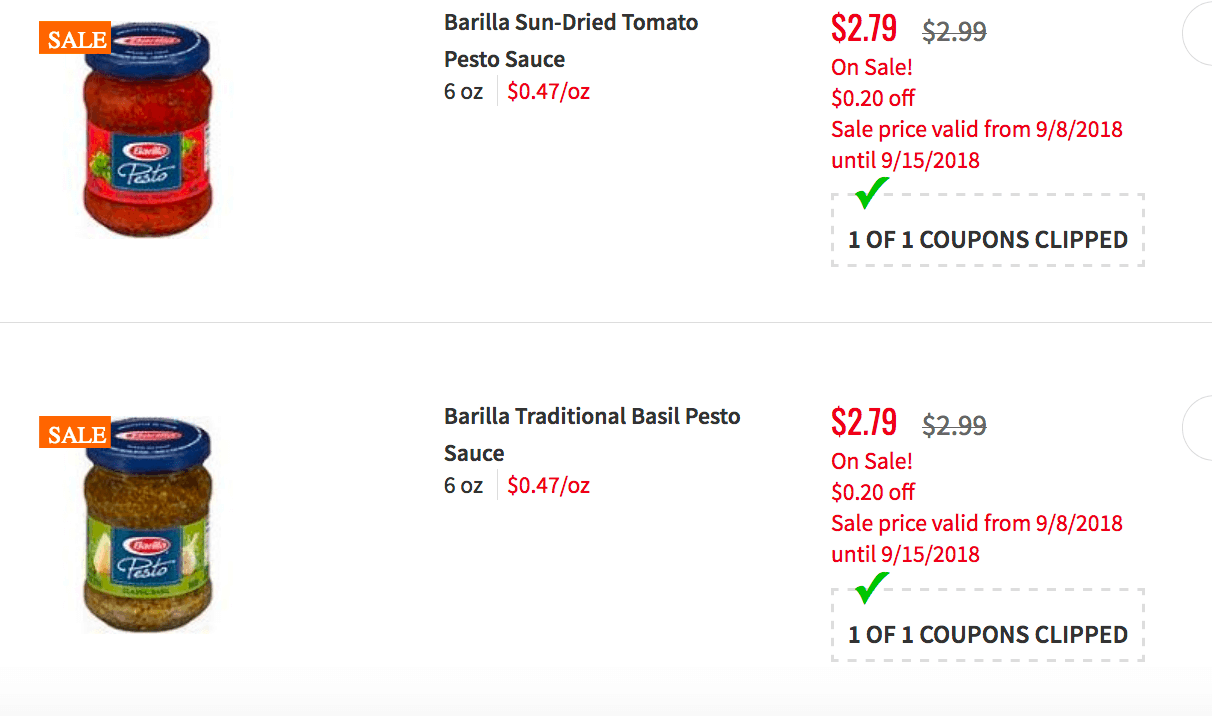The image depicts a webpage featuring a detailed view of two product listings for sauces, aimed at online shoppers considering these options. 

Located at the top left is a jar of sun-dried tomato pesto sauce. The vibrant red sauce is encased in a jar, prominently labeled "Sale" with an orange and white sticker. The product, specified as "The Ariella Sun-Dried Tomato Pesto Sauce," comes in a 6-ounce jar priced at 47 cents per ounce. The sale price is clearly marked in red font: $2.79, reflecting a 20% discount from its original price of $2.99. The sale is valid from September 8, 2018, to September 15, 2018. A small green check mark indicates that one coupon has been clipped for this item.

Below this, there is another jar on display, labeled similarly with a red, orange, and white "Sale" sticker. This jar contains a "Traditional Basil Pesto Sauce," also in a 6-ounce size and priced at 47 cents per ounce. Like the previous item, it is on sale for $2.79, marked down from $2.99, valid from September 8, 2018, to September 15, 2018. The caption notes that a coupon has been clipped for this product as well.

This webpage provides a well-organized, clear presentation of discounted sauces, complete with pricing details, sale durations, and coupon statuses, making it convenient for shoppers to make informed decisions.